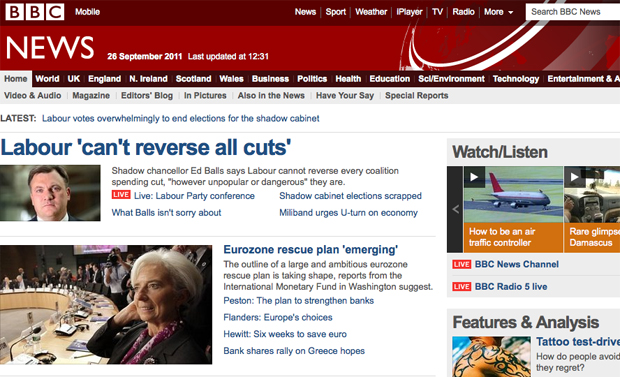Screenshot of BBC News Homepage

The screenshot captured is a view of the BBC News homepage. At the very top, a deep red-brown horizontal rectangle hosts the BBC logo on the left. Each letter of "BBC" is situated inside a white square box, and the letters are in the same rust red-brown color as the background. To the right of the logo, the word "mobile" is displayed.

On the far right of this top bar, there is a white menu bar featuring several navigation options, including "News," "Sport," "Weather," "iPlayer," "TV," and "Radio." A drop-down menu labeled "More" follows these options, and a white search bar is on the extreme right with the placeholder text "Search BBC News."

Below this top section, a prominent red rectangle displays the label "NEWS" on the left, with the current date and last updated time noted alongside it. Underneath this, another menu bar lists categories such as "Home," "World," "UK," "England," "Ireland," "Scotland," "Wales," "Business," "Politics," "Health," "Education," "Science," "Environment," "Technology," and "Entertainment."

Further down, a grey menu bar provides additional navigational links. Directly beneath it, on the left side, is the headline section. The first headline, marked in blue with a small accompanying image, reads "Labour votes overwhelmingly to end elections for the Shadow Cabinet." 

A light blue line separates this headline from the next, which is displayed in larger blue text, stating "Labour can't reverse all cuts." This article features a photograph of a man, serving as a headline tagline.

Another article appears below, featuring a smaller picture on the right side with the blue headline text "Eurozone rescue plan emerging."

To the right side of the screen, there are media options with clickable videos labeled "Watch" and "Listen," offering users access to audiovisual content.